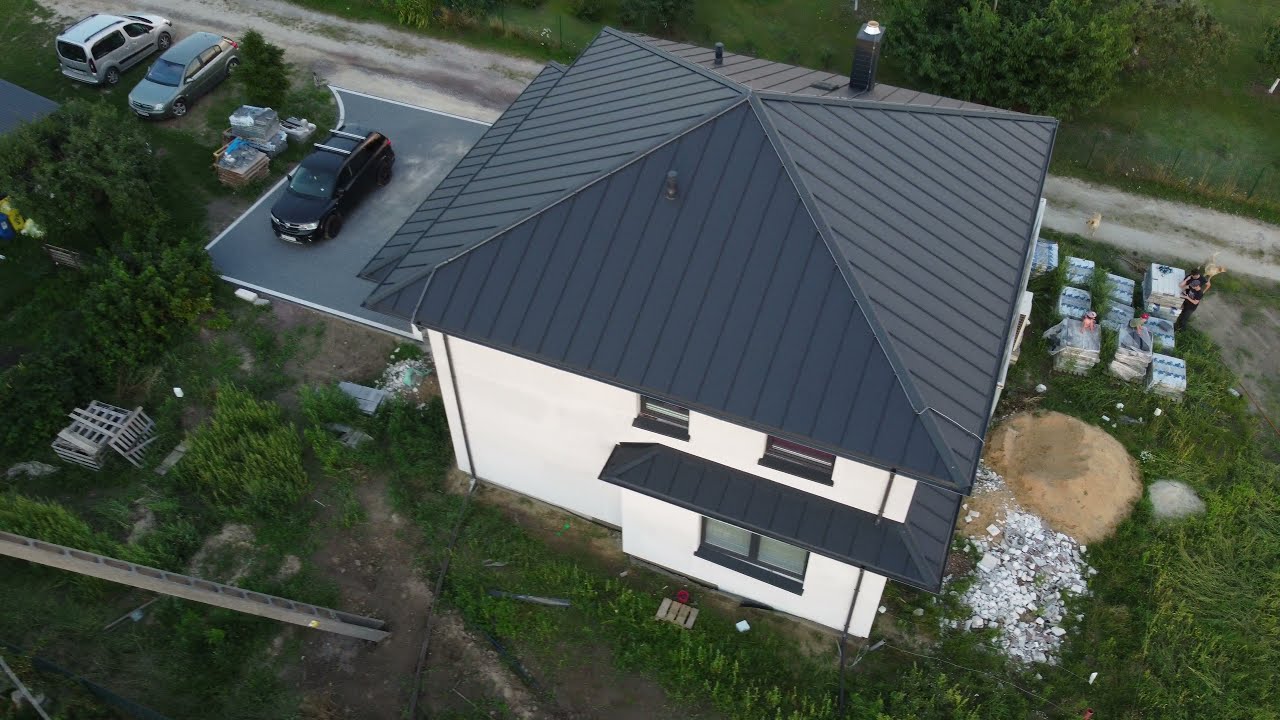This aerial photograph, likely taken from a drone, showcases a two-story white house with a dark gray, if not black, metal pyramidal roof. The roof features several vents and is complemented by a matching metal awning wrapping around at least two corners of the structure. The surrounding yard appears somewhat cluttered, suggesting ongoing construction or renovation. To the left of the house, a gray paved driveway accommodates a black SUV, with two additional cars, a hatchback sedan and a silver van, parked on a dirt section nearby. On the right side of the property, there is a considerable mound of beige sand and various stacks of construction materials, including white boxes, crates, and a ladder. Green grass, trees, and bushes surround the house, with a small gravel road extending across the back of the property. This detailed scene highlights both the architectural features of the house and the bustling, construction-heavy environment in its vicinity.